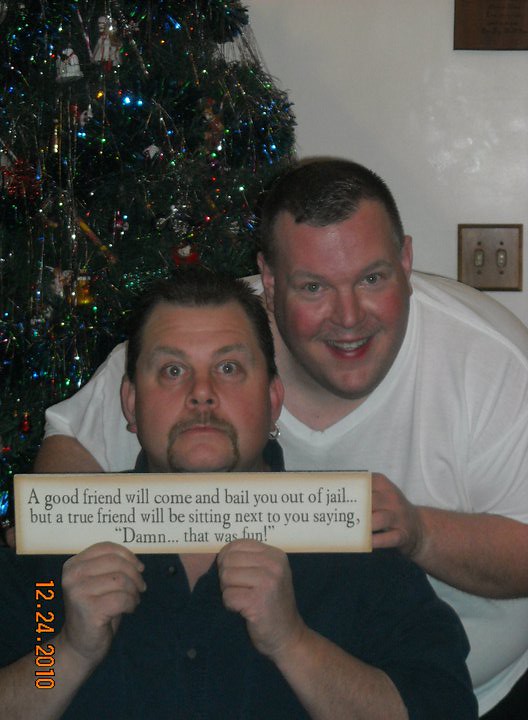The photographic image captures an indoor scene during Christmastime in a house. Two men are the subjects of the photo; a white, overweight man in a white t-shirt stands smiling with his hands resting on the shoulders of a bearded and mustached man who is seated. The seated man, also white, sports a serious or stunned expression and wears a black shirt. He holds a sign that reads, "A good friend will come and bail you out of jail, but a true friend will be sitting next to you saying, 'Damn, that was fun.'" In the background, a Christmas tree decorated with ornaments is visible, along with a framed picture on the wall. The date "12.24.2010" is watermarked in orange letters on the lower left part of the image.